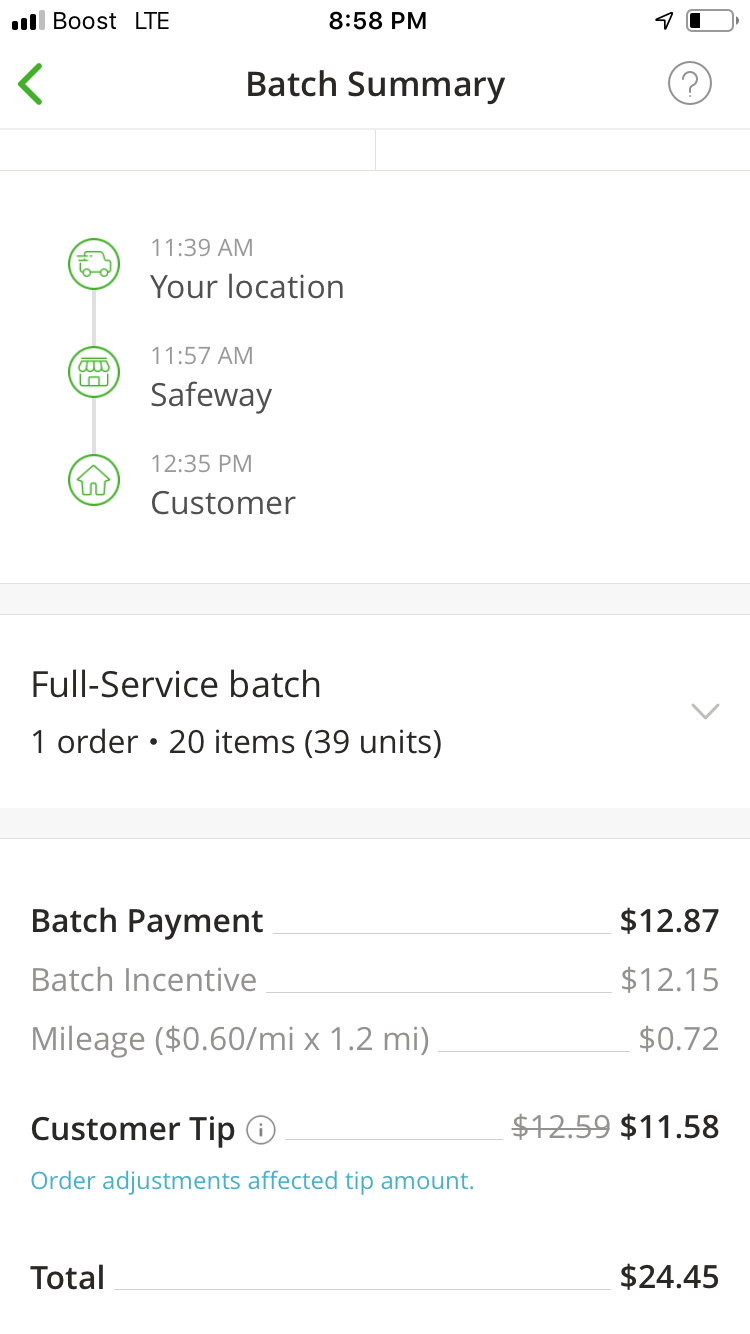**Caption:**

A detailed screenshot from a mobile phone displaying a bulk purchase summary. At the top of the screen, the status bar shows the phone's battery life in the top right corner and the LTE signal with "Boost" in the top left corner. Centered is the time, 5:58 p.m., followed by a bold heading titled "Batch Summary." 

Below the heading, there is a green arrow on the left and a circled question mark on the right. The interface then depicts a progression of steps with time stamps and icons: 

1. 11:39 a.m. – A car icon indicating the starting location.
2. 11:57 a.m. – A house icon representing a stop at Safeway.
3. 12:35 p.m. – Another house icon marking the final delivery to the customer.

Below this timeline, there is a gray bar labeled "Full Service Batch - 1 order of 20 items (30 units)." To the right of this text, a drop-down box offers additional details.

The next section, separated by another gray bar, lists payment information. "Batch Payment" is highlighted in bold, showing $12.87. Below it, "Batch Incentive" is listed with a smaller greyed text noting $12.15. Mileage compensation is calculated at $0.60 per mile times 1.2 for a total of $0.72.

Customer tip details are provided next, showing a $12.59 tip, with a note about order adjustments affecting the tip. The total amount earned, highlighted in bold and positioned at the far right, is $24.45.